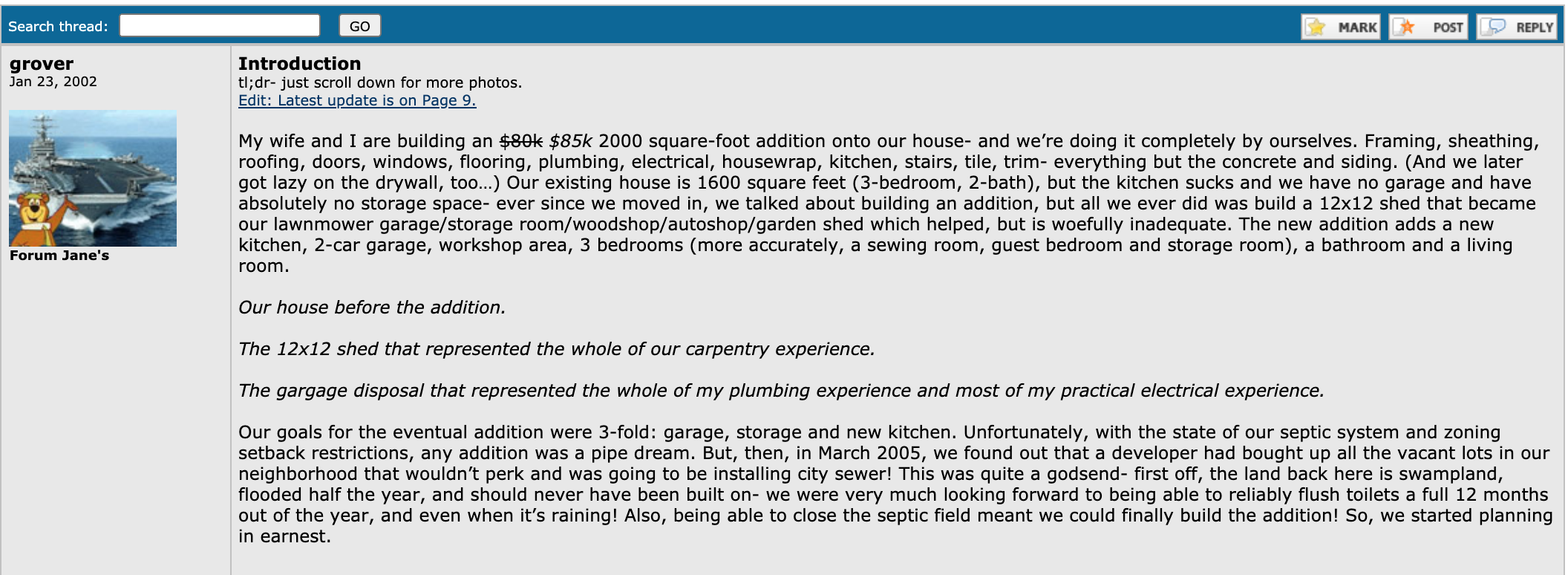This image is a screenshot of an online forum post created by a user named Grover on January 23rd, 2002. The forum interface features a light gray or light blue background that suggests an older website design. Grover's profile picture appears to be an image of a military carrier ship with a superimposed graphic of Yogi the Bear. The post, located to the right of the profile picture, is notably lengthy and is titled "Introduction" at the top. In the top right corner of the post, three selectable buttons are visible: "Mark," "Post," and "Reply." The overall aesthetic of the forum indicates an antiquated online platform.